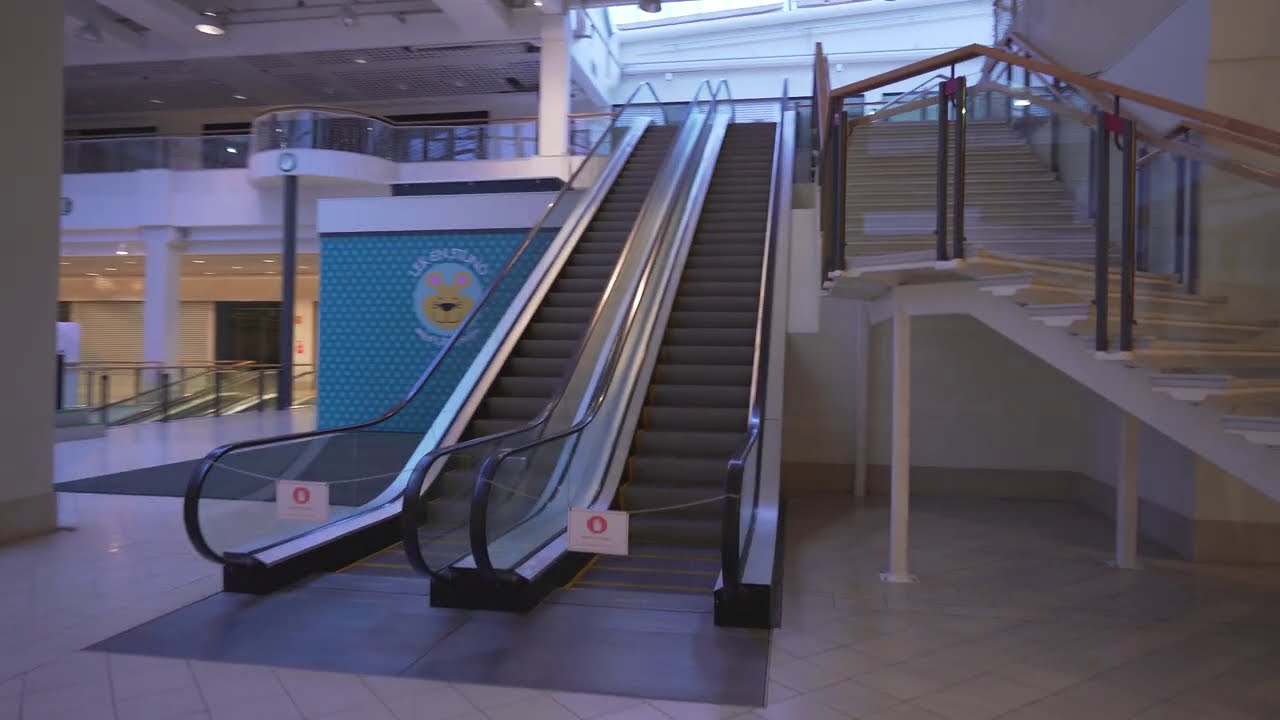The photograph captures the interior of an apparently deserted shopping mall. Dominating the scene are two adjacent escalators, each with gray metal steps and black handrails, flanked by glass panels. Both escalators, positioned centrally in the image, are visibly out of service, adorned with unreadable yet distinctly cautionary white signs. To the immediate right, there is a staircase that extends partly beyond the image frame, featuring white-painted steps and brown wooden handrails. The mall's floor is covered in polished white ceramic tiles, contributing to the overall sterile atmosphere.

In the background, on the left side, a blue wall adorned with a whimsical cartoon bear logo in gold, black, and pink is set against a teal and light blue polka-dot backdrop. Above and below this logo, faint white text can be discerned, adding an element of curiosity. Further into the background, several closed shop fronts are visible, with their blacked-out windows contributing to the sense of emptiness. A high ceiling supported by white concrete pillars and dotted with numerous lights stretches overhead, adding to the vast, open feel of the space.